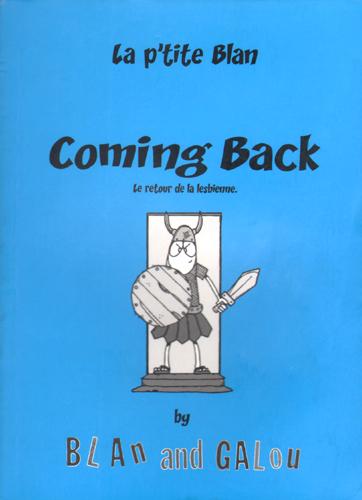The book cover features a light blue background with multiple lines of black text. At the top, it reads "La Petite Blonde," followed by "Coming Back," and "La Retour de la Lesbienne." Beneath the text is a detailed black and gray drawing of a Viking standing in a doorway. The Viking, appearing fierce and determined, is depicted with a conical helmet adorned with horns, glasses, and is holding a sword in their left hand and a wooden shield with nails on the edges in their right hand. The Viking is dressed in a black pleated skirt, black armor, and sandals, standing on black steps. Below the drawing, more black text reads "Bye," and finally, "Blonde and Gallo." The illustration and text suggest themes of resilience and return, framed in a stylistic, possibly satirical, manner.